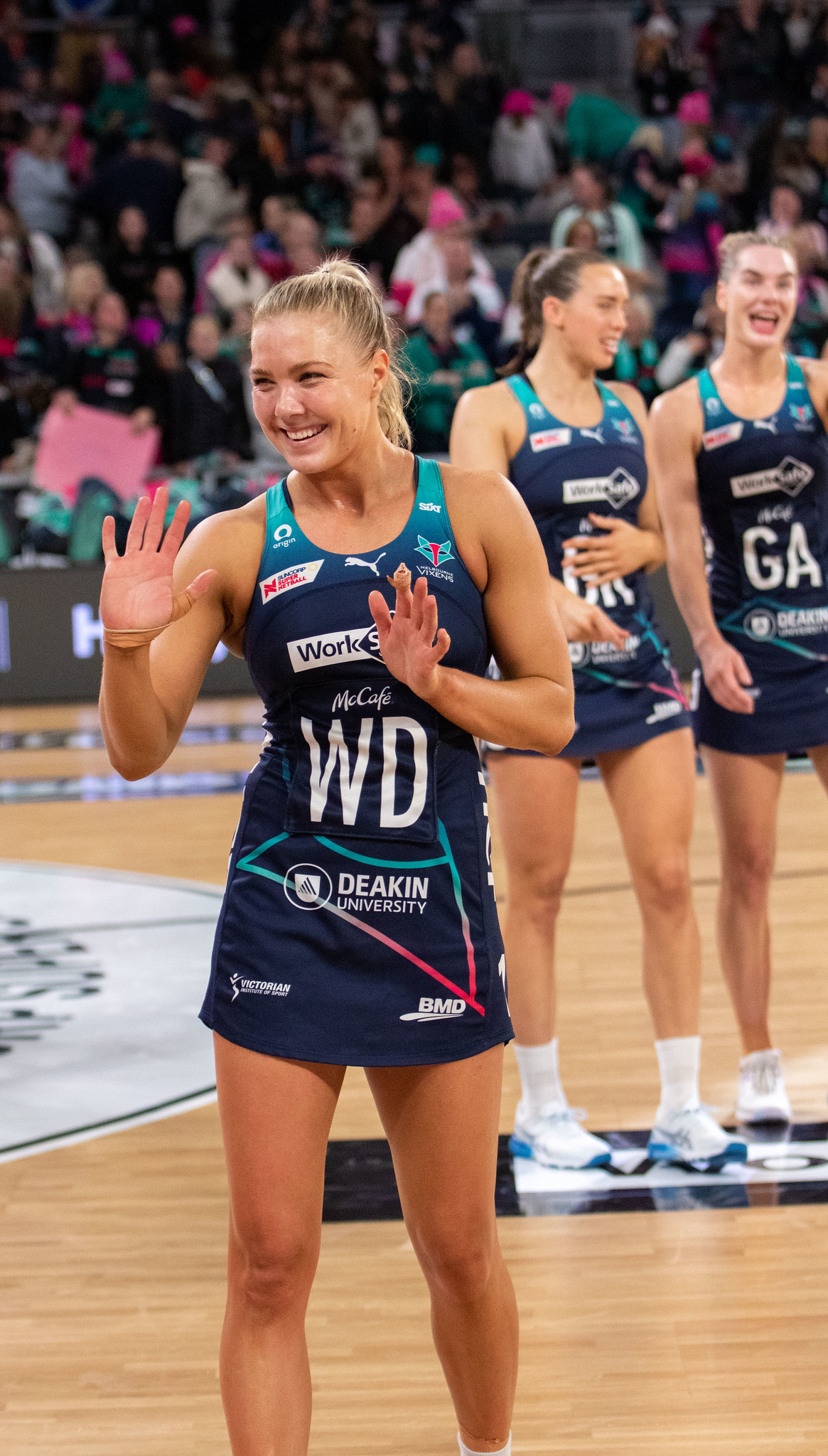The image features three female basketball players standing on a polished wooden court, identifiable by the partial circular half-court symbol visible. The focal point is a smiling player in the foreground with blonde hair tied in a ponytail. She is wearing a navy blue tank top and skirt ensemble with "Deakin University" and a McCafe logo, along with the initials "WD" prominently displayed on her jersey. Her hands are extended outward, her demeanor cheerful. Behind her are two other players, similarly attired, engaging in a conversation and also smiling. The background shows a blurred audience, filled with spectators, some of whom are wearing bright pink hats, adding to the vibrant atmosphere within the gymnasium.